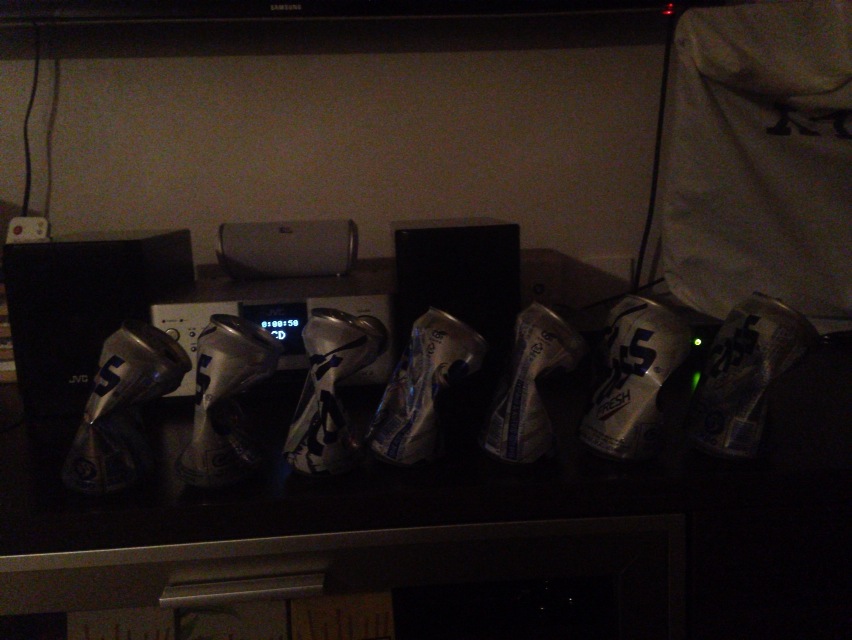In this dimly lit indoor color photograph, a detailed scene emerges. The focal point is a stereo system with illuminated blue numbers, indicating that it is turned on. The stereo, adorned with a smaller gray speaker on top and flanked by two black JVC speakers, rests on a TV stand or tabletop. In the foreground, seven pop cans, all bearing the word "fresh," stand upright in a slightly slanted position to the right. Each can appears to be crushed in the middle, as if compressed by hand, and they are neatly aligned side by side. The subdued lighting gives the image a slightly mysterious ambiance, drawing attention to the peculiar arrangement of crushed cans in contrast to the organized audio equipment behind them.